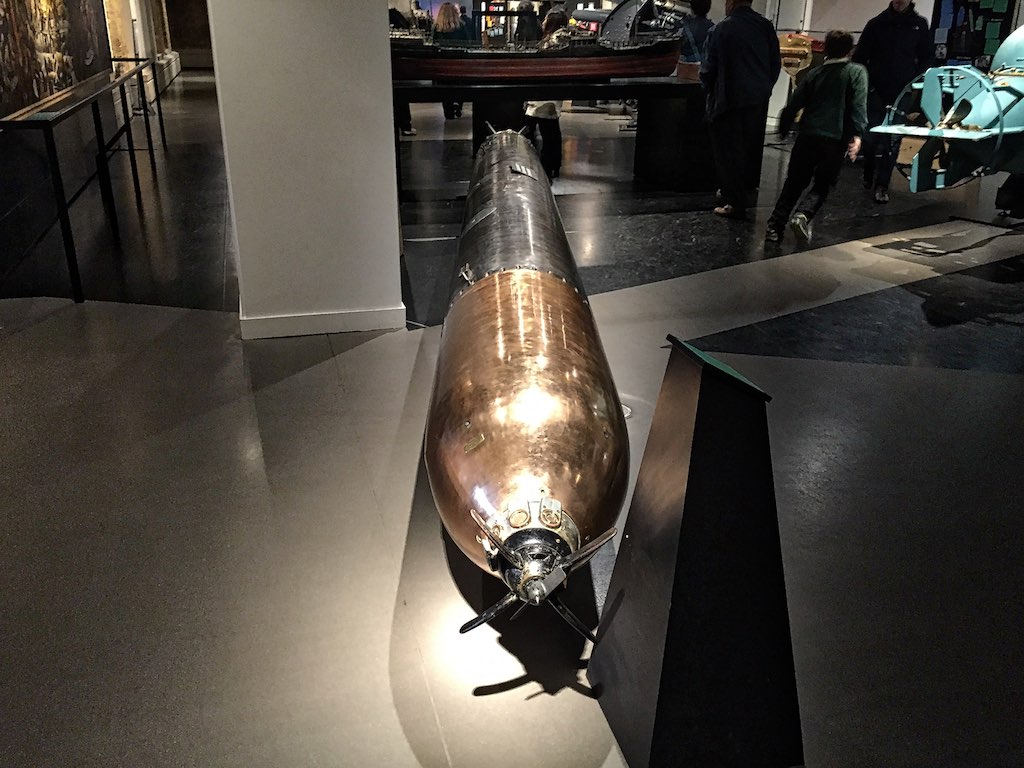This image captures the inside of a museum showcasing a central highlight—a black and gold torpedo or missile prominently displayed. The torpedo, possibly launched from a submarine, features four propeller blades at the back. The scene unfolds on a black and white floor, and to the right, there is a light blue, propeller-equipped underwater capsule, appearing rideable. In the mid-ground, an older-style ship model is visible, suggesting a maritime or nautical theme to the exhibit. The setting includes various other models and displays, with visitors perusing the exhibits predominantly on the right side. To the left, a long, thin table stands unadorned, adjacent to a wall featuring a picture or display. The dominant colors in the scene are white, gold, black, and light blue, creating a balanced and visually engaging environment.